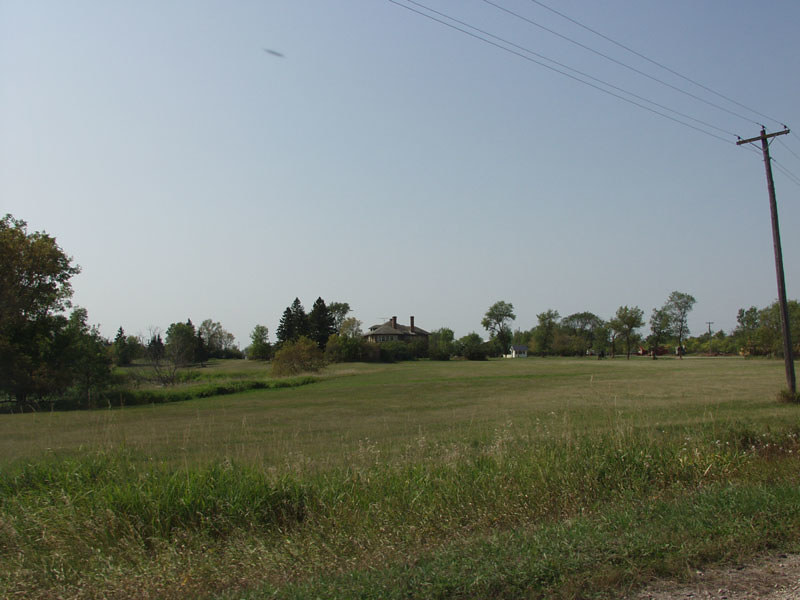In this image, we're looking at a distant view of a large residential house set far back, possibly taken from the side of a road. The house, which may have multiple chimneys, is situated in the middle of a vast open field. The field is divided into two sections: the area closest to the camera features high, unmaintained grass, while the section closer to the house appears meticulously mowed and flat, with a slight gentle slope. The scene is framed by tall trees scattered on either side of the house, as well as around a smaller white building with a gray roof to the right of the main house. The sky is a light blue, with no visible clouds, indicating perhaps an overcast evening or dusk rather than a bright sunny day. Power poles and electrical wires are visible, reinforcing the inference that the photo is taken from a roadside perspective. The overall atmosphere of the image is serene and quiet, capturing the expansive, open land around the residential property.